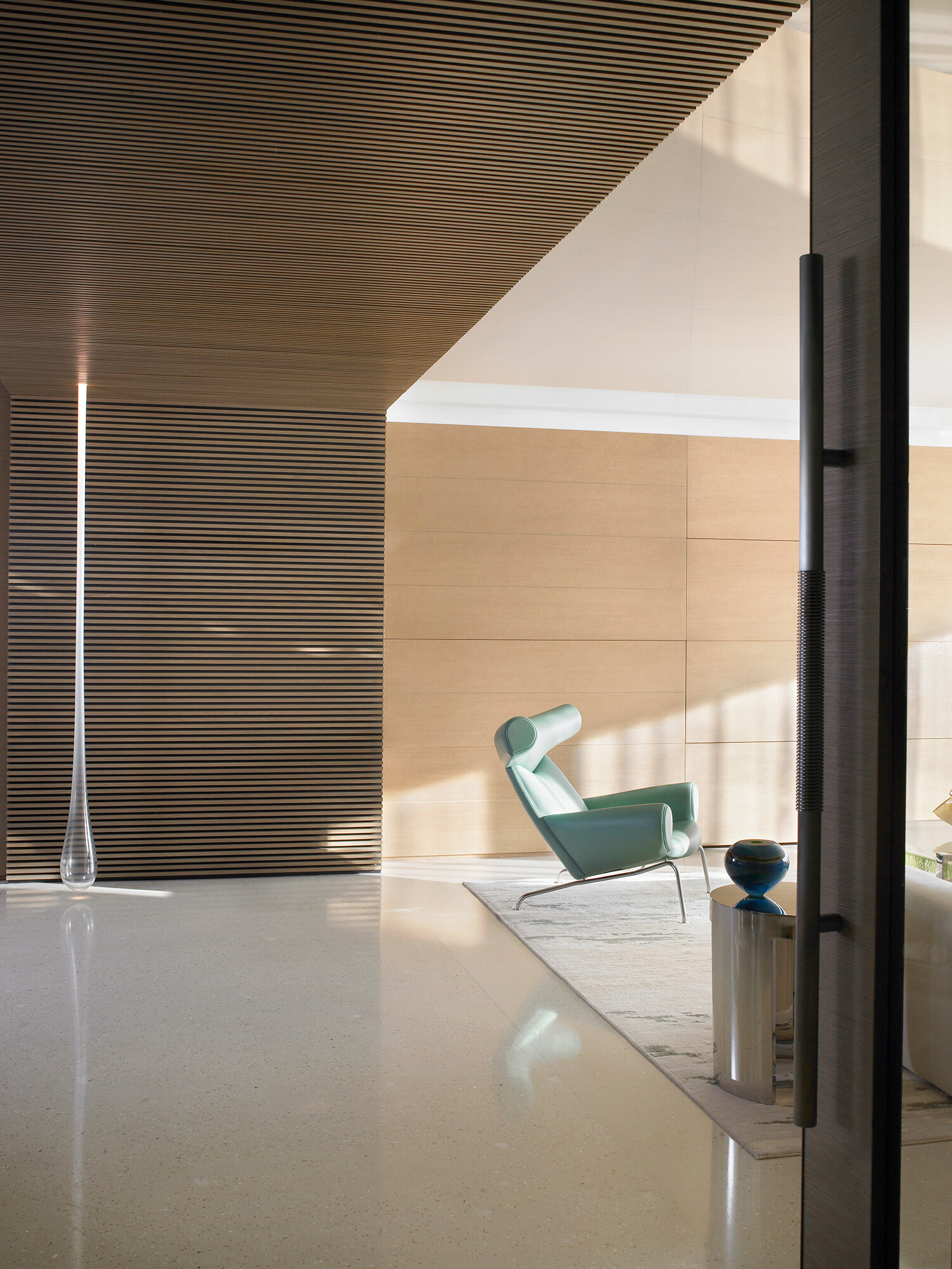This image, a 3D color illustration created in an app like SketchUp, portrays a modern, contemporary living room viewed from a hallway through a transparent glass door with a long black handle on the right side. The room features a white rectangular carpet adorned with gray abstract patterns, situated on a beige speckle stone floor. A distinct aqua-upholstered modern chair, slightly bent with an overstuffed neck roll and an angular silver base, stands prominently near the top left corner of the rug. Adjacent to the right side of the chair is a partially visible white sofa. To its left sits a round, chrome-colored modern table topped with a green vase. On the left side of the room, there's a foyer area characterized by a horizontal slat wall and ceiling treatment made from beige wood. This space is accentuated by a tall, teardrop-like glass sculpture reaching from the floor to the ceiling, resembling a large drop of water with light at its apex. Additional elements such as part of a table and a lamp are partially visible, contributing to the modern aesthetic of the room.